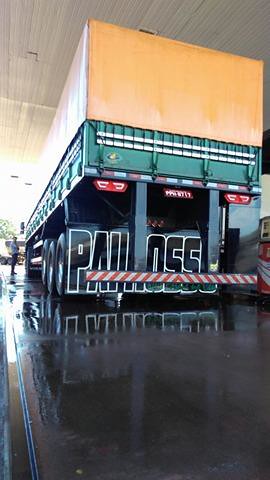This vertical photo captures an industrial-sized green truck from the rear, situated in what appears to be a loading or truck depot. The wet ground, potentially from recent rain or cleaning, reflects the ambient light, adding a sleek appearance to the scene. The truck's top is covered with an orange tarp, adding a contrasting element to its otherwise utilitarian look. The wheels, visible on the left side, are black with gray or silver rims, and the truck sits on a black frame adorned with red lights and a red-and-white safety bar at the bottom. The rear of the truck features partially obscured text starting with "P.A.I" and ending with "O.S.S." A man, possibly the driver, stands near the driver's side door, far in the distance, emphasizing the truck's immense size and the high vantage point of the photo.